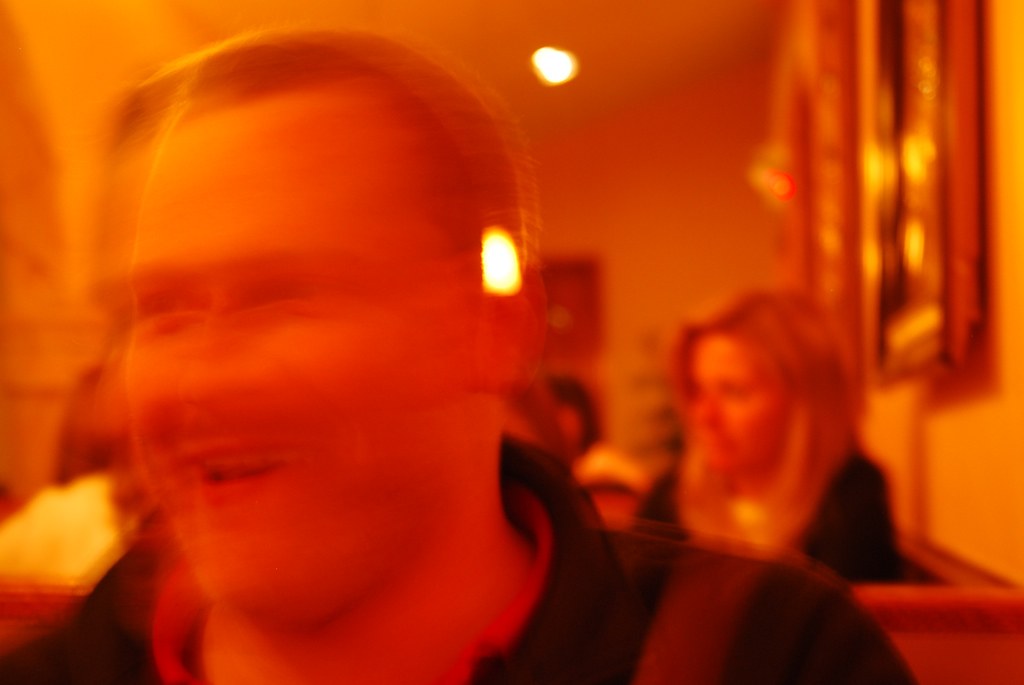The photograph features a person in the foreground, seemingly captured mid-motion, which has resulted in a blurred, doubling effect around his head, giving the image a dynamic quality. He has short, light-colored hair and is smiling subtly. He is dressed in black and red clothing. Behind him, a partial view of a booth is visible, along with several seated individuals. There are gold objects adorning the wall in the background and overhead lights visible. Over his shoulder is a woman with long blonde hair, wearing a dark shirt. The background includes additional people, adding context to the scene. The overall image has a slightly grainy texture, enhancing its candid and spontaneous feel.